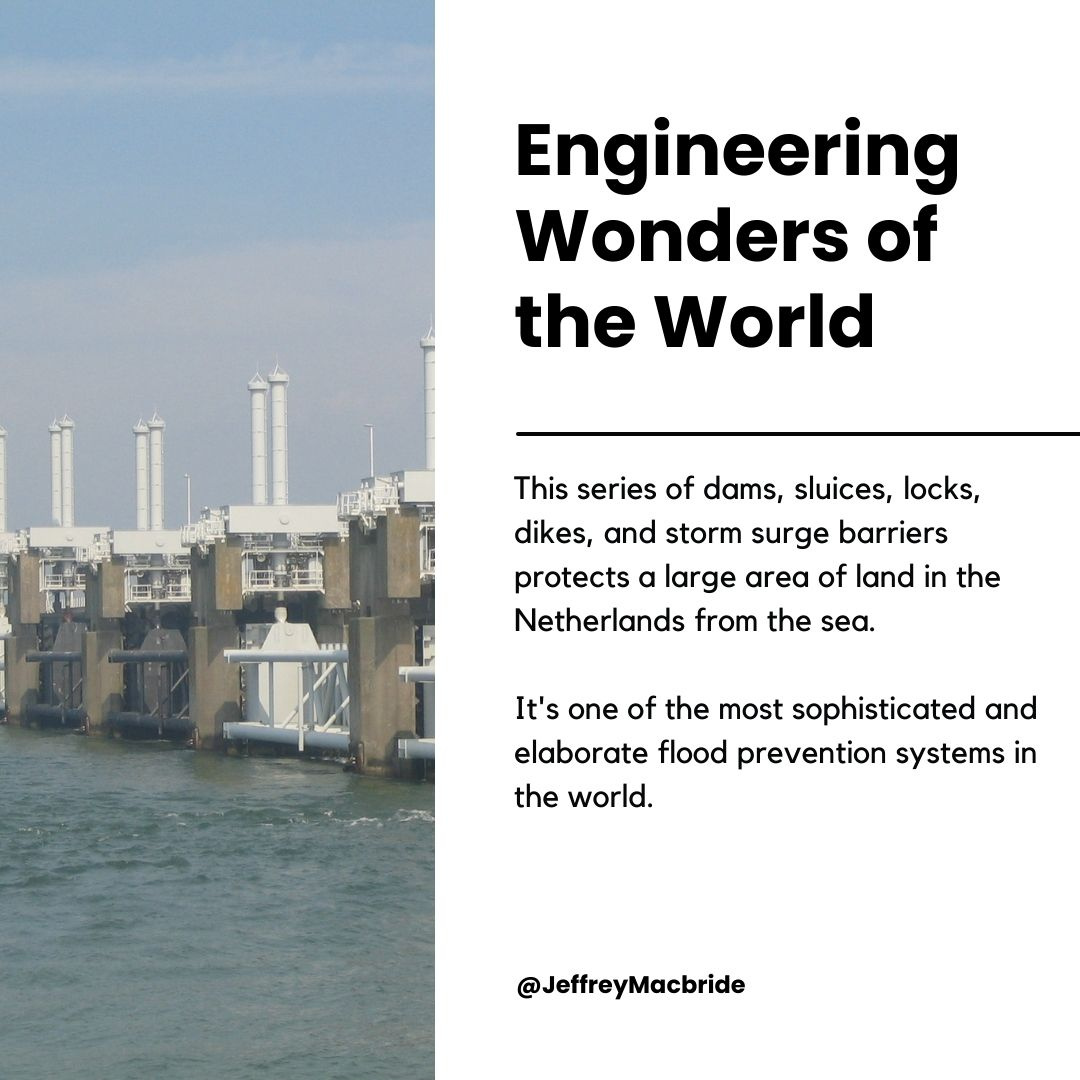This page, potentially from a magazine, highlights an engineering wonder of the world, described in black text. The central image depicts a water system, likely in the Netherlands, featuring a dam with large white stacks on top, under a blue sky. This structure, with its distinct white roofs and little vanities in between, resembles square arches floating on the water. To the right of the image, a detailed paragraph titled "Engineering Wonders of the World" explains that this series of dams, sluices, locks, dikes, and storm surge barriers protects a large area of land in the Netherlands from the sea. It is noted for being one of the most sophisticated and elaborate flood prevention systems in the world. The text is credited to Jeffrey McBride, with a line underneath the title and all letters in black.